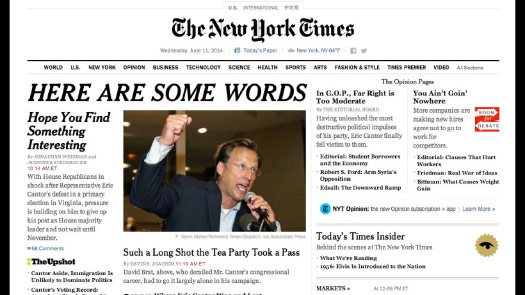A New York Times snippet captures the tension following Representative Eric Cantor’s unexpected defeat in a Virginia primary election, leading to growing pressure for him to relinquish his role as House Majority Leader ahead of November. Accompanying the article is a poignant image of a man, likely Cantor, dressed in a suit coat and white button-down shirt, raising a fist while holding a microphone—his tie notably absent. The headline emphasizes the internal strife within the GOP, summarizing that the far-right faction, which Cantor once emboldened, has now turned against him. An inset highlights another issue: companies increasingly requiring new hires to agree not to work for competitors. The snippet also includes a teaser for the Times Insider section, promising a behind-the-scenes look and curated reading recommendations, though the full content is cut off.